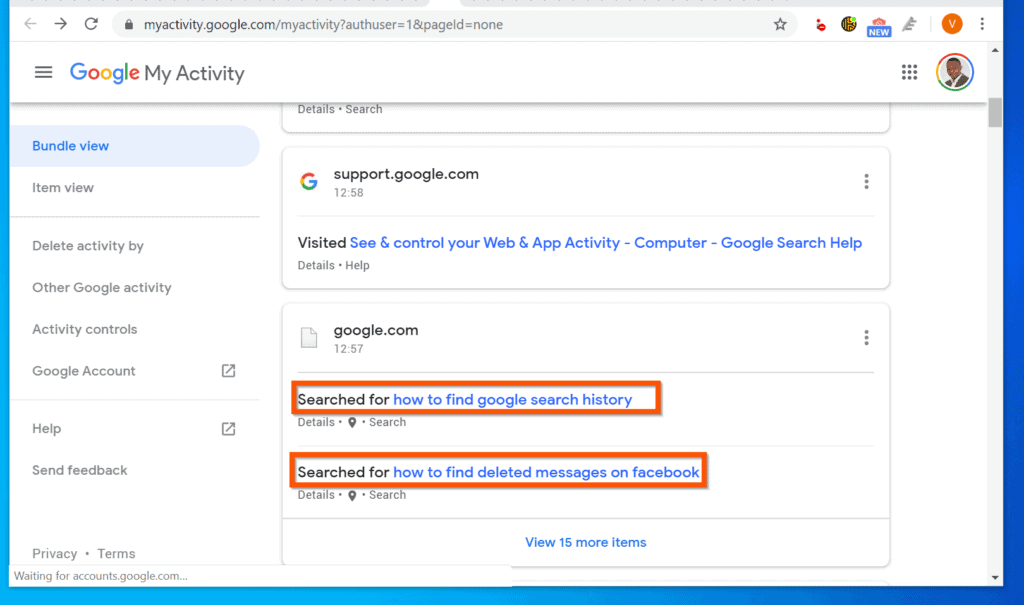**Caption:** 

This image is a detailed screenshot of the Google My Activity settings page, viewed in the Chrome browser. At the top of the Chrome window, the traditional navigation buttons are visible: a back arrow, a forward arrow, and a refresh icon. Following these, the address bar displays the URL "myactivity.google.com/myactivity?offuser=18&pageId=none," with a clickable five-pointed star at the end for bookmarking the page. To the right of the URL are various Chrome extension icons.

Below the address bar, a white navigation header reads "Google My Activity." On the left-hand side, a vertical menu lists several options: "Bundle view" (currently selected), "Item view," "Delete activity by," "Other Google activity," "Activity controls," "Google account," "Help," and "Send feedback." To the right of this menu, the main content area shows the "Bundle view" interface, which starts with a section summarizing recent activity. At the top of this content area is a box with "support.google.com," indicating that the user has visited this support page. Below that, additional text reads, "See and control your web and app activity - Computer - Google Search Help."